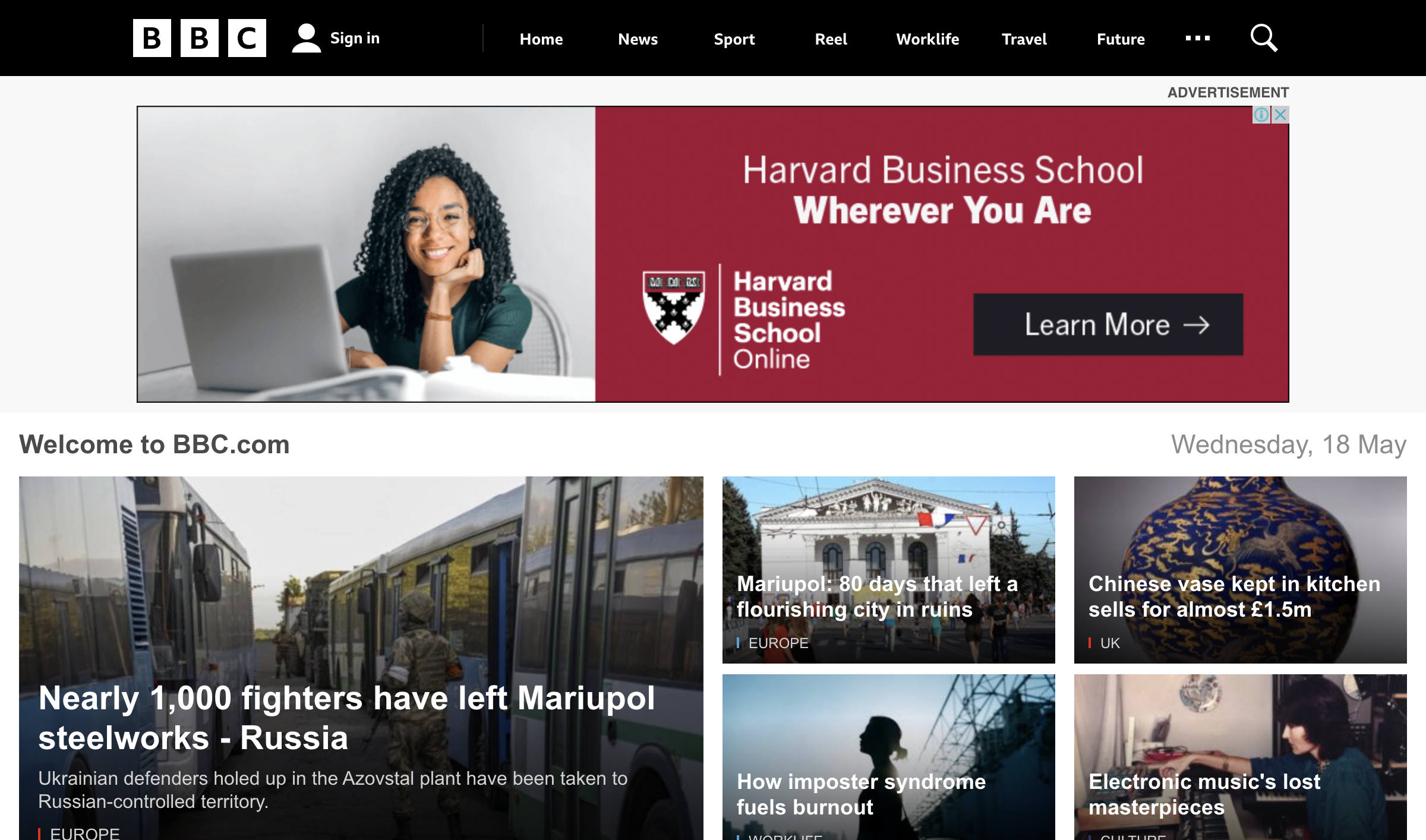The image is a screenshot from the BBC website. At the top, the distinctive BBC logo is prominently displayed, featuring three white squares each containing a capital letter "B," "B," and "C" in bold black lettering, all housed within a black rectangle. Adjacent to the logo is a simplistic user profile icon resembling a circle for the head and a semicircle for the shoulders, accompanied by the "Sign In" option. 

To the right of this, the navigation menu is listed horizontally, starting with "Home," followed by "News," "Sport," "Reel" (spelled R-E-E-L), "Worklife," "Travel," and "Future." Furthermore, the menu includes three horizontally aligned white dots and a white magnifying glass icon for search functionality.

Beneath the navigation bar, an engaging image features an African American woman seated at her desk with an open laptop. She is wearing glasses, smiling warmly, and has a head of dark, curly hair. She rests her head on her hand, propped up by her elbow on the desk, and is seated in a gray chair.

Next to her image, a red box prominently displays the text "Harvard Business School—Wherever you are," with an accompanying black box labeled "Learn more." At the bottom of the image, there are five clickable thumbnail pictures, each leading to additional content.